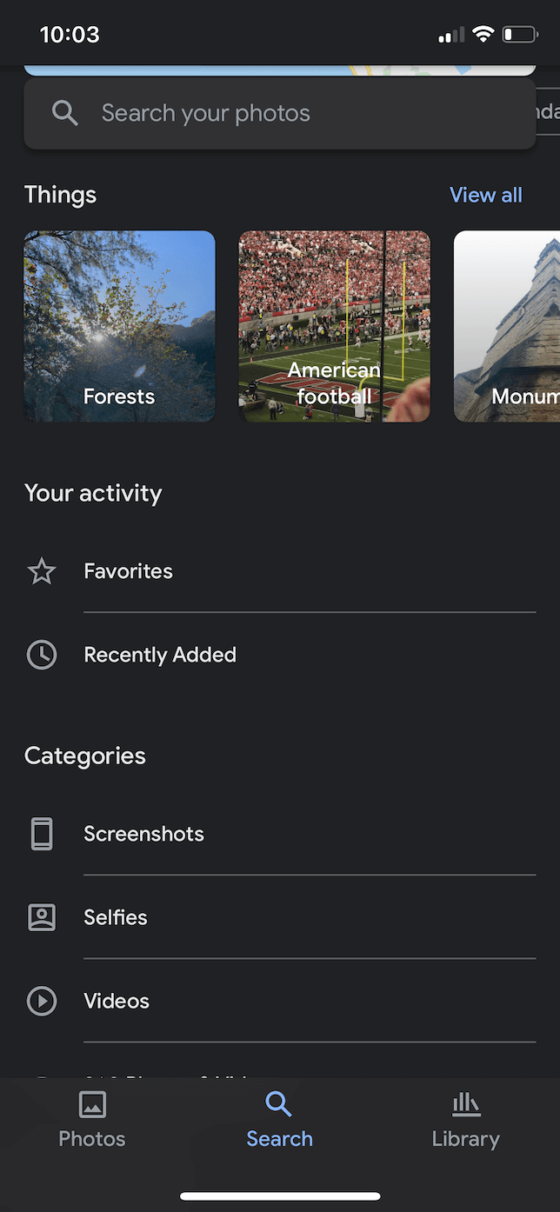This image, taken from a smartphone, displays a vertical, rectangular interface, characteristic of a photo gallery application. The time '10:03' is shown at the top, followed by a long blue line beneath it. Directly below, there is a search bar containing the placeholder text 'Search your photos'. At the very top, the section labeled 'Things' appears in white text.

This section highlights three thumbnails. The first thumbnail shows trees and the sky with the label 'Forests'. The second thumbnail depicts a large crowd of people seated in a stadium, likely for an American football game. The third thumbnail features a gray monument with the label 'Monument'.

Underneath these thumbnails, there are sections labeled 'Your Activity', 'Favorites', and 'Recently Added'. As the interface scrolls down, a 'Categories' section appears, featuring a thumbnail labeled 'Screenshots' beside it.

Directly below, another thumbnail is labeled 'Selfies'. Adjacent to this, a circular icon with a right-pointing arrow is labeled 'Videos'. Towards the bottom of the screen, there is a rectangular section for 'Photos' and above it, a blue magnifying glass icon with the word 'Search' written in blue text. Finally, an image of the side of some books is labeled 'Library' at the bottom of the screenshot.